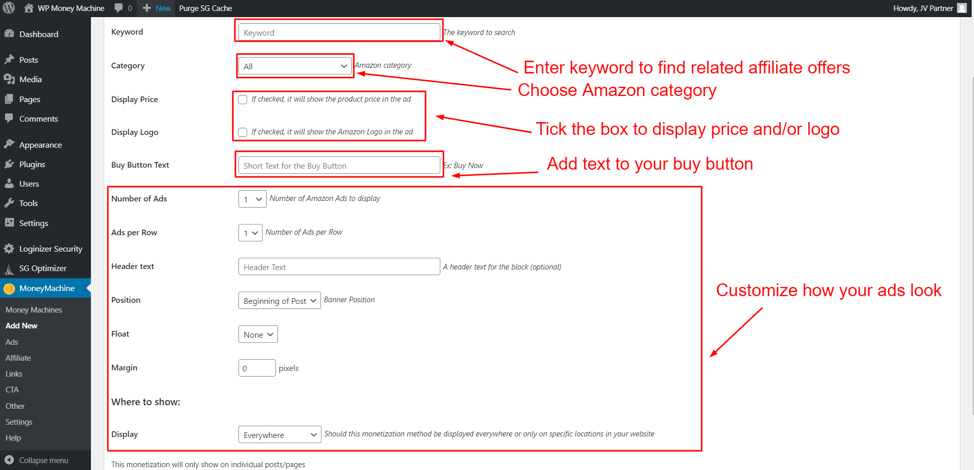Here is a cleaned-up and detailed caption for the image described:

---

The screenshot appears to be from a webpage related to affiliate marketing, specifically focusing on managing affiliate orders and monetization. The interface is predominantly set against a white background, except for the left-hand sidebar, which features a black to dark gray gradient.

On the right side of the screen, various interactive elements are highlighted with red outlines. Each of these boxes includes descriptive text followed by an arrow pointing towards them. From the top:

1. Two small red-outlined boxes are accompanied by arrows leading to text that reads: "Enter keyword to find related affiliate offers" and "Choose Amazon category for this."
2. Below these, there is a larger box, similarly outlined in red, with an arrow pointing to it. The accompanying text states: "Tick the box to display price and/or logo."
3. Further down, another red-outlined box of similar size to the first two has text with an arrow indicating: "Add text to your buy button."
4. The largest box on the screen is also outlined in red, with the text: "Customize how your ads look."

On the left-hand sidebar, a vertical menu lists various sections of the website, including Dashboard, Posts, Media, Pages, Comments, Appearance, Plugins, Users, Tools, and Settings. Additionally, there is an option labeled as SG Optimizer. The active section, marked in a light sky-blue shade to indicate selection, is labeled as "Money Machine." This highlights the current focus of the screen on managing and optimizing affiliate monetization tools.

---